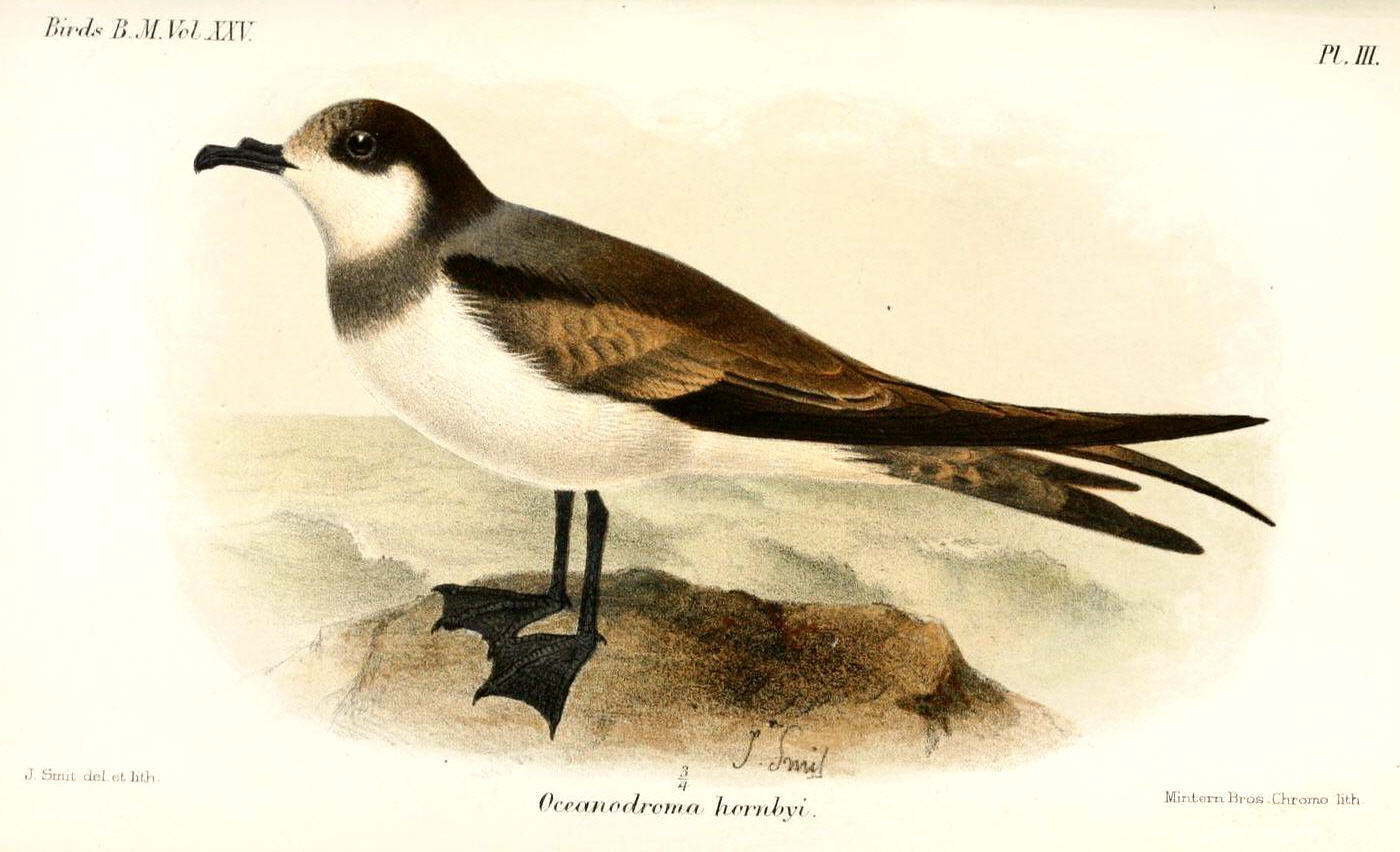The image features a meticulously hand-drawn bird, primarily rendered in neutral tones including brown, black, off-white, and hints of yellow. The bird is depicted standing on a rock with the backdrop resembling ocean waves. It has a black beak, black feet, and showcases a white chest and chin. The image includes text in several locations: in the top left corner, it reads "Birds BM Volume XXV," and in the top right, "PLIII." The lower left corner contains faint text, likely the signature "J Strutt Del et HTH," and the bottom center displays the bird’s scientific name, "Oceanodroma hornbyi." The bottom right has indistinct text due to faintness. The artistic style and educational context suggest that this drawing, possibly done with watercolors or fine pencils, might be part of a reference book.